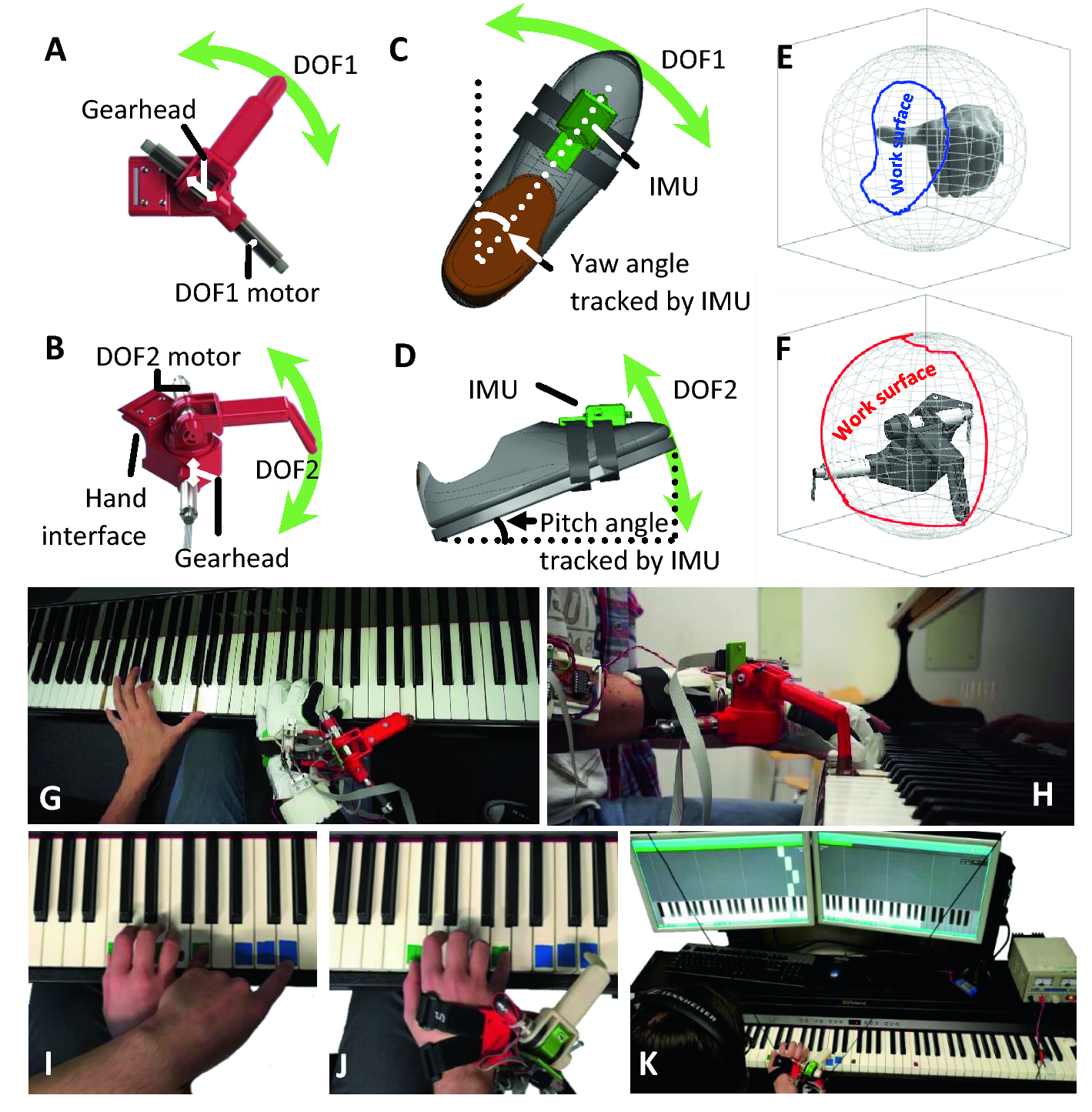This image is a large, detailed square diagram split into an upper and lower section. The top part features six small images against a white background labeled A through F, arranged in two columns and three rows: A above B, C above D, and E above F. Each image displays various components of a robotic or music-related device alongside green two-way arrows indicating movement or interaction. The upper left image (A) shows a red and gray "gear head" with a "DOF-1 motor," while the image below it (B) presents another part of the device. The central column (C and D) includes images of a shoe, depicting both an outline and a side view with a "tracked by IMU" label highlighting the pitch angle. The upper right images (E and F) display other elements related to this system.

The lower part of the image comprises five photographs of a piano keyboard labeled G through K. These images offer various perspectives, including close-ups of the keys and shots of a hand on the keys. Notably, the hand appears to be using the device from the upper left image (A) during its interaction with the keyboard. The final two shots also show green computer screens displaying a keyboard at the bottom, further indicating interaction between the device and the musical instrument. The diagram overall suggests a robotics system that tracks and assists in playing a keyboard, likely involving both hand and foot components.